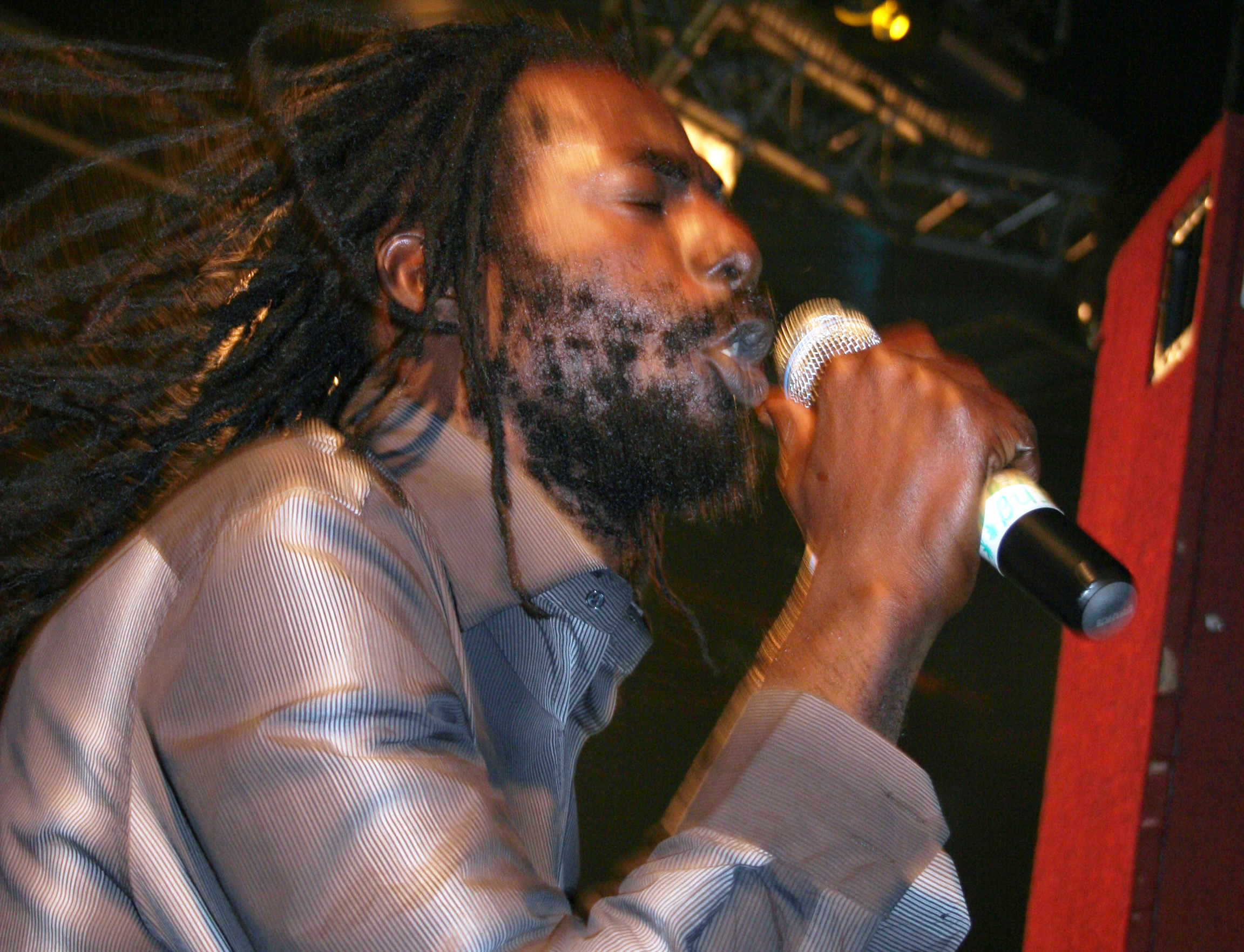An African-American male singer is captured mid-performance. His long, black braided hair is dramatically flying towards the left corner of the image, enhancing the dynamic nature of the scene. The singer sports a beard and mustache, adding to his distinguished appearance. He is dressed in a striking lavender jacket with subtle, white stripes, which appears to be crafted from a silky material. Holding a white microphone to his mouth, he seems deeply engrossed in his singing, evidenced by the expressive look on his face. The background features a steel structure that likely forms part of the stage setup, illuminated by a light from the top right. To the singer's left stands a tall wooden speaker with a square opening at its top, adding to the authenticity of the live performance environment.